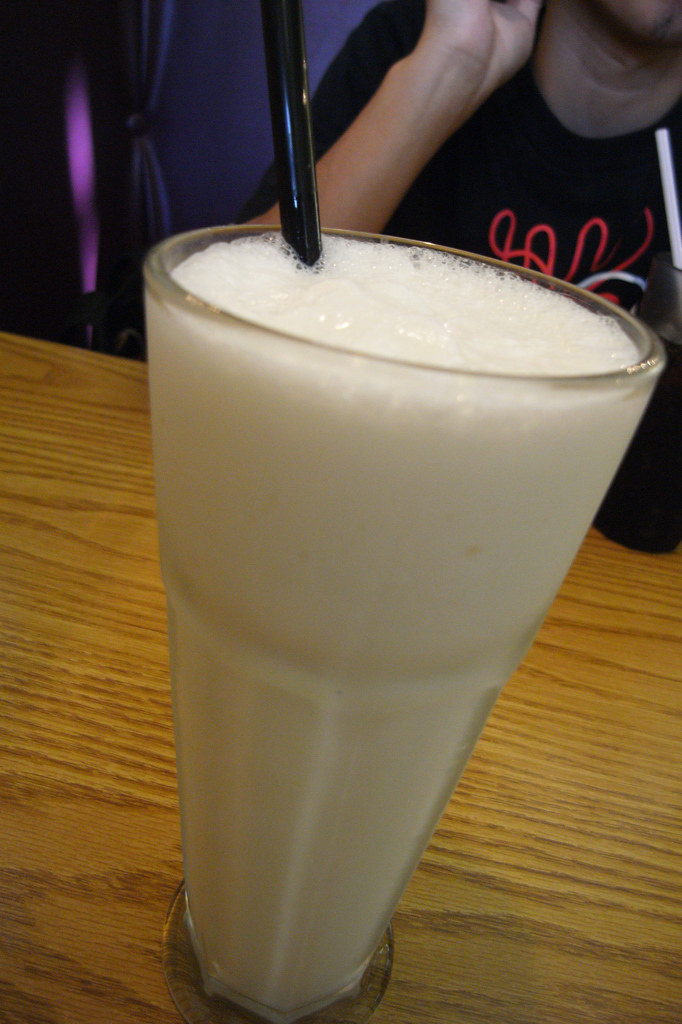This photograph captures a creamy, white milkshake served in a tall, diner-style glass, occupying about three quarters of the image from a top-down vantage point. The milkshake is perched on a semi-gloss wooden table that reflects a touch of sheen. A black straw pierces through the frothy surface of the milkshake. Behind the glass, there is a human figure clad in a short-sleeved black shirt adorned with red squiggly or cursive lines. The person’s arm is raised towards their chin, although only the neck and collar area are visible. In the background, a deep purple wall and what might be a purple curtain or ornament add a splash of color, with a lighter purple vertical line subtly contrasting in the shadows. To the right, the edge of the photo hints at another glass with a straw, possibly containing a darker beverage like cola.